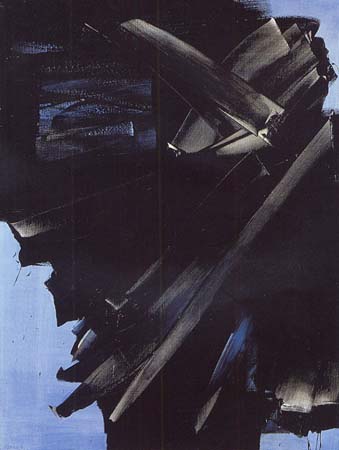This painting, titled *Pienter 23, Avril 1963* by Pierre Soulages, is a striking abstract modernist work rendered in oil on canvas. Set against a predominantly azure blue background, the composition features a collection of dark gray and black metallic elements that appear corroded and are arranged in a complex, irregular stack. This structure, reminiscent of sharp implements such as swords or knives, extends diagonally from the top left to the bottom right of the portrait-oriented canvas. The metallic elements form a partial teepee-like shape, with one prominent piece slanted across the top, seemingly unsupported by the others. The lower right and upper left corners of the painting reveal more of the blue background, providing a stark contrast to the dense, fragmented forms in the center. The interplay of light and shadow enhances the silvery appearance and sharp edges of these objects, making the overall image both compelling and enigmatic.